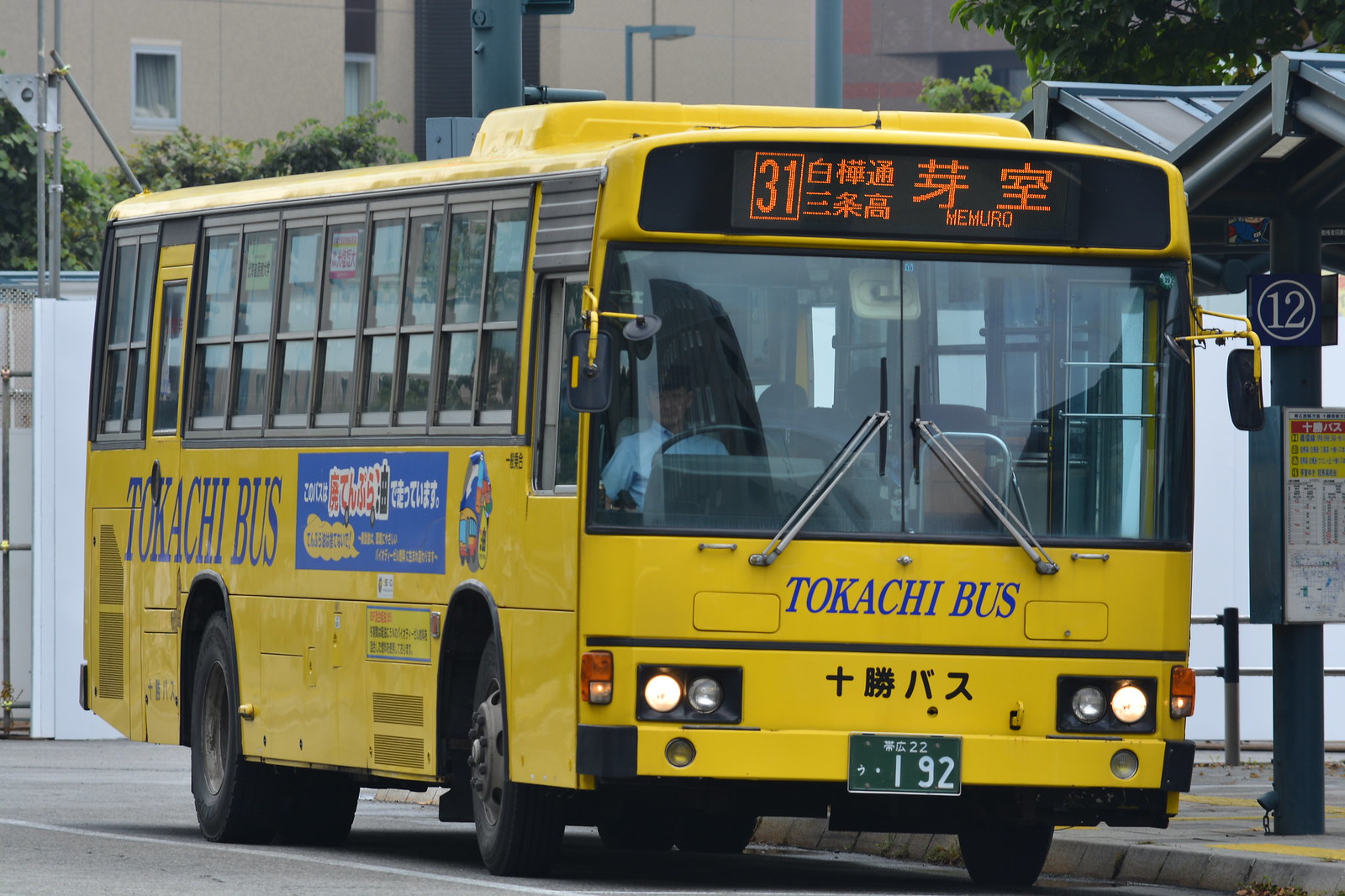In this vibrant image, a bright yellow Tokachi bus, likely located in Japan, is prominently displayed. The bus features distinctive Japanese characters on both the front and side, with "Tokachi Bus" clearly labeled. The front of the bus includes a black banner displaying the number "31" and other orange characters, as well as a license plate showing characters followed by "22" and the larger number "192." The bus is currently stationed at bus stop 12, a covered area that shields passengers from the elements. Beneath the bus stop sign, there is what appears to be a bus schedule. A blue advertisement with building icons and additional text in Japanese decorates the side of the bus. In the background, a multi-story building looms, and a white wall can be seen beyond the bus stop. The driver is visible on the left side, and the bus has a row of windows and a yellow rear door for passenger exit. The overall scene suggests a busy urban environment where the bus is preparing to collect passengers.